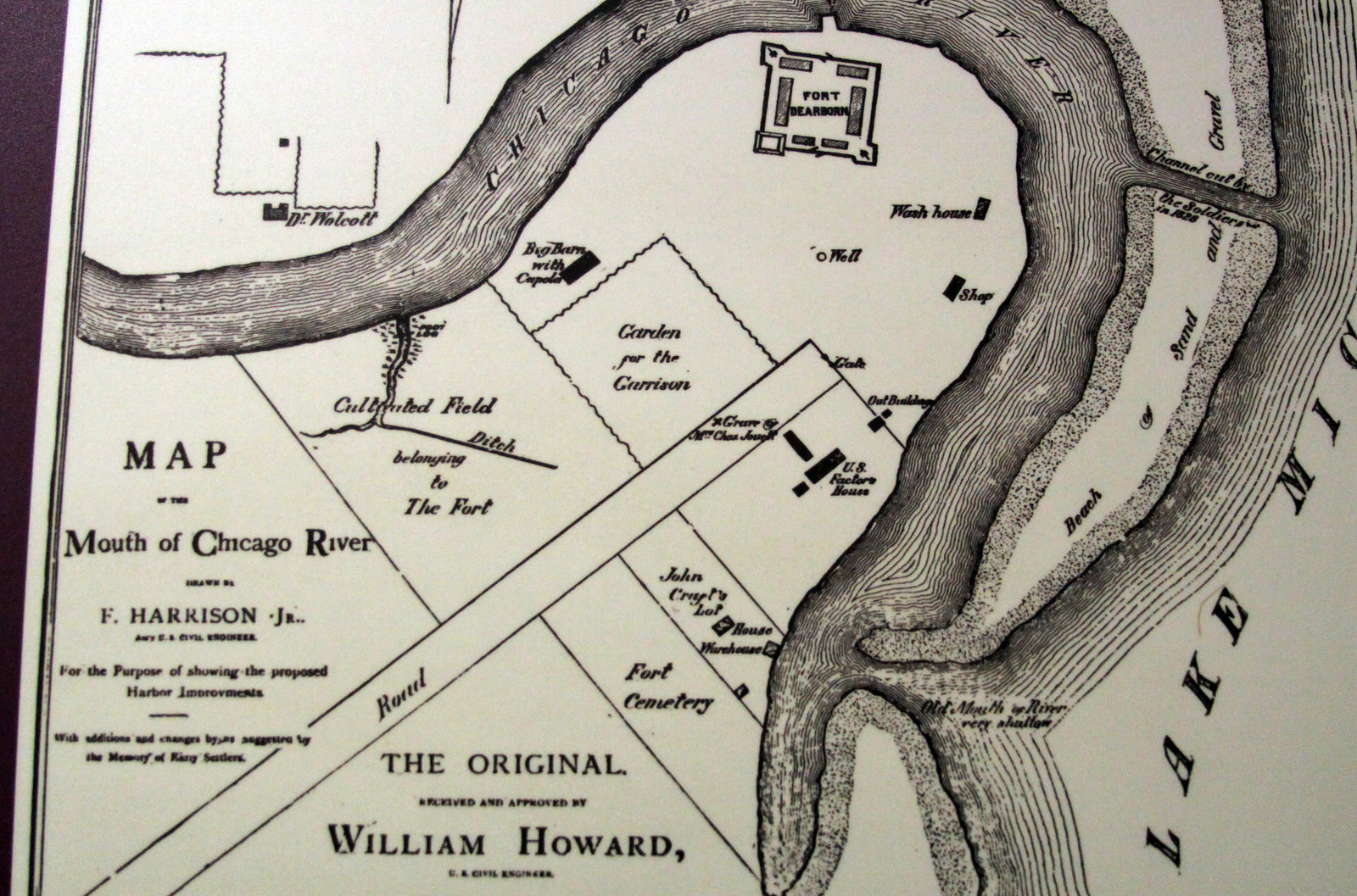This image showcases a historical, ivory-colored map with a distinctive black sketch illustrating the mouth of the Chicago River. Central to the map is the winding Chicago River, depicted in bold contrast, while intricate, smaller labels adorn the surrounding features. Notably, near the river bend, the map marks Fort Dearborn, a significant landmark. Additional annotations detail various structures and areas, including a well, wash house, shop, outbuilding, U.S. factor house, garden for the garrison, cultivated field, and a fort-associated ditch.

The bottom left-hand corner of the map references “The Original by William Howard” and notes his role as a U.S. civil engineer. The map bears the inscription, "Map of the Mouth of the Chicago River," credited to F. Harrison Jr., described as being created for the purpose of illustrating proposed harbor improvements. This text indicates the map's historical value, reflecting changes and plans from its era, making it both a visually interesting and informative artifact of early Chicago.